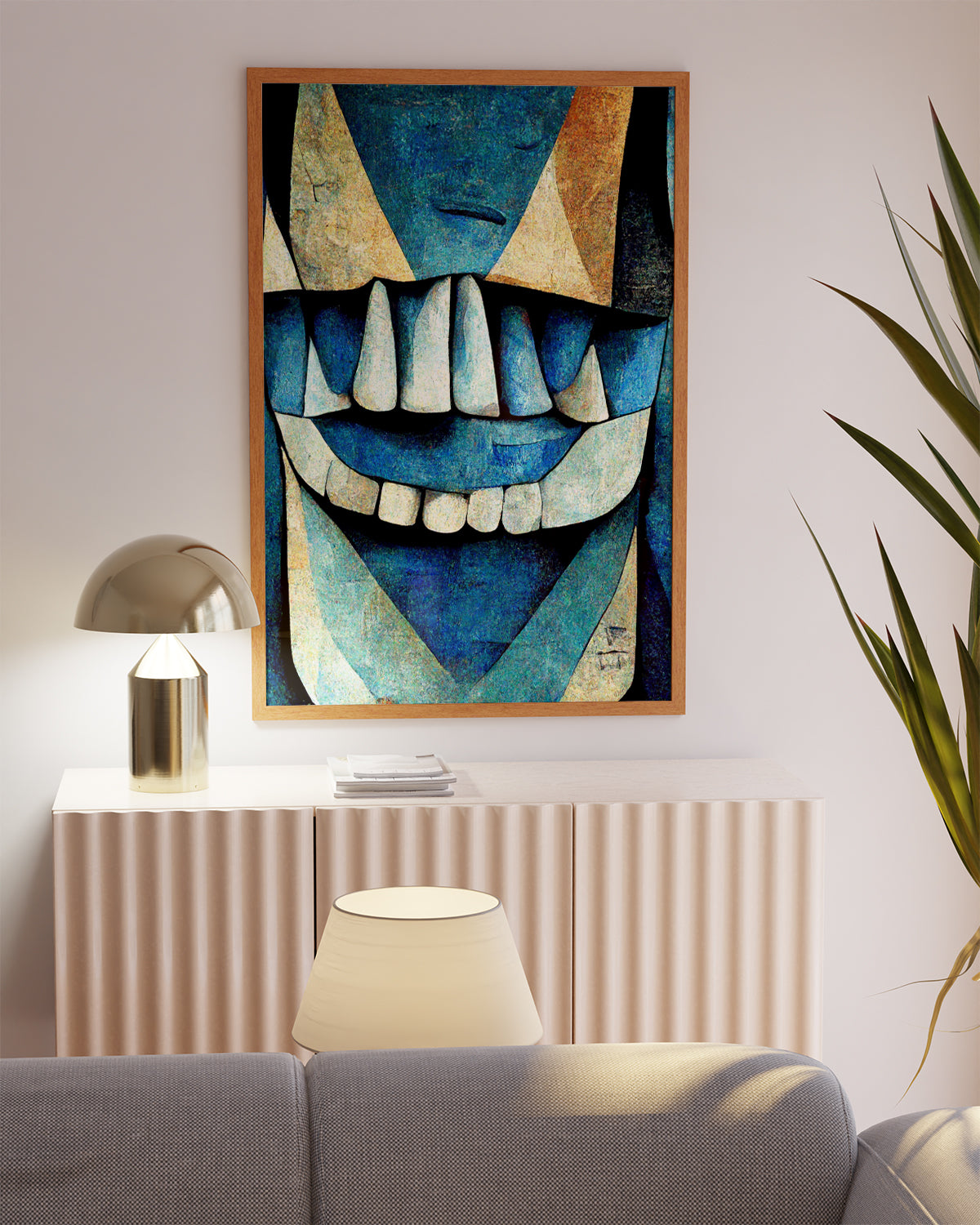The photograph depicts a well-lit living room with sunlight streaming in from the right side, suggesting it was taken in the late morning or early afternoon. The focal point is a large, colorful artwork centered on a soft off-white wall. The artwork is housed in a brown rectangular frame and features a greenish-blue background with two light brown triangular shapes at the top, resembling an abstract face. Beneath these shapes are rows of white and bluish teeth-like structures, adding a geometric complexity to the piece.

Below the painting sits a white credenza with corrugated panels. On the left side of the credenza is a bronze-colored lamp with a pencil-thin base and a hooded, semi-circular top. A stack of unopened mail rests in the center of the credenza. 

In front of the credenza, partially obstructing it, is a light gray fabric couch. Behind the couch, on the right side, stands another lamp with a linen shade. Adjacent to this setup, a potted plant extends its thin green stalks into the frame, adding a touch of nature to the indoor scene. The overall composition combines vibrant artwork with practical living room elements, creating a cozy yet artistic atmosphere.